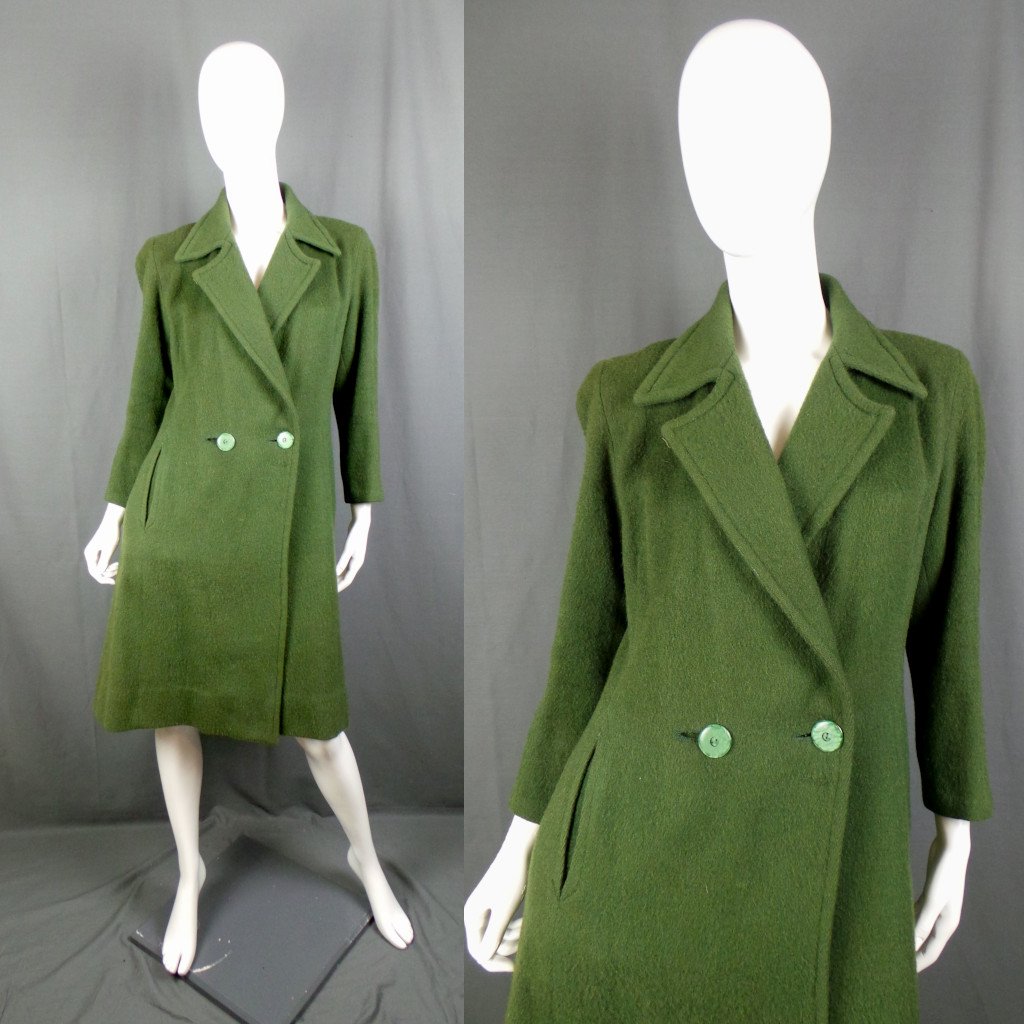The image is a product photograph featuring a white mannequin, positioned against a gray cloth backdrop that also covers the floor. There are two panels in the image: the left panel shows a full-body view of the mannequin, while the right panel provides a closer, more detailed view of the upper body. The mannequin is dressed in a women's knee-length overcoat, which is a moss green color with large, distinct kelly green buttons. The coat features a notch collar and buttons around the stomach area. The mannequin itself has a featureless head, contributing to a stark, artificial look in comparison to its hands and legs.